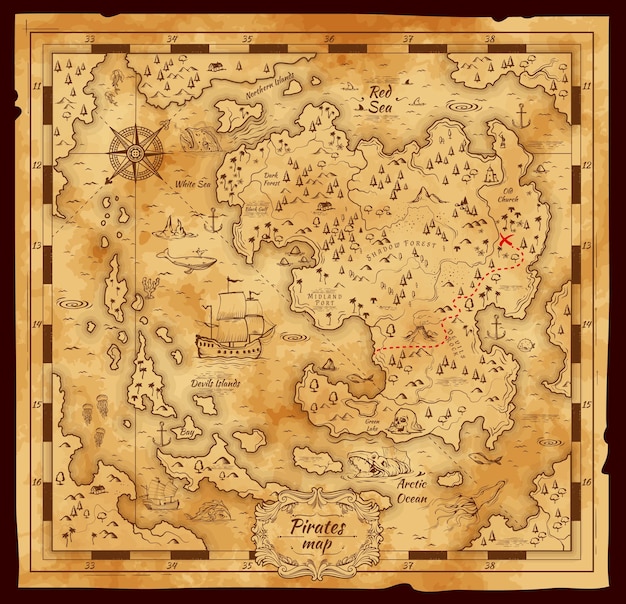This detailed pirate map is a richly illustrated, brown and cream-hued artifact, bordered in brown and marked with a multitude of intriguing details. At the bottom, the title boldly states "Pirate's Map." The map depicts a larger landmass to the right, encircled by various smaller islands on the left, all amidst swirling tones reminiscent of aged parchment. The text "Arctic Ocean" appears in fancy print towards the bottom right.

To the top left is a compass rose, and just to its right, the map names the "White Sea." Above the compass, at the very top, it declares the "Northern Islands," while the "Red Sea" is noted in the upper right section. The map features diverse, fantastical sea creatures including a squid, a spouting whale, and a large-headed beast in the waters, enhancing its maritime theme.

In the center, an old pirate ship with white sails navigates near "Devil's Island," a designated area to the lower left. A red dashed line snakes its way from the southern part of this island, heading east through indistinct terrain and past "Devil's Rock," before winding northeast to a red "X" marking the treasure's location. Above this treasure spot, the old church is drawn and labeled.

Anchors and other maritime motifs are scattered across the map. Significant landmarks, such as the "Red Sea" positioned on the upper right and the labeled "White Sea" further south, demarcate the fictional world. This treasure map, complete with a trail of red dots leading to the iconic "X marks the spot," conjures a sense of adventure and hidden riches, an embodiment of pirate folklore.